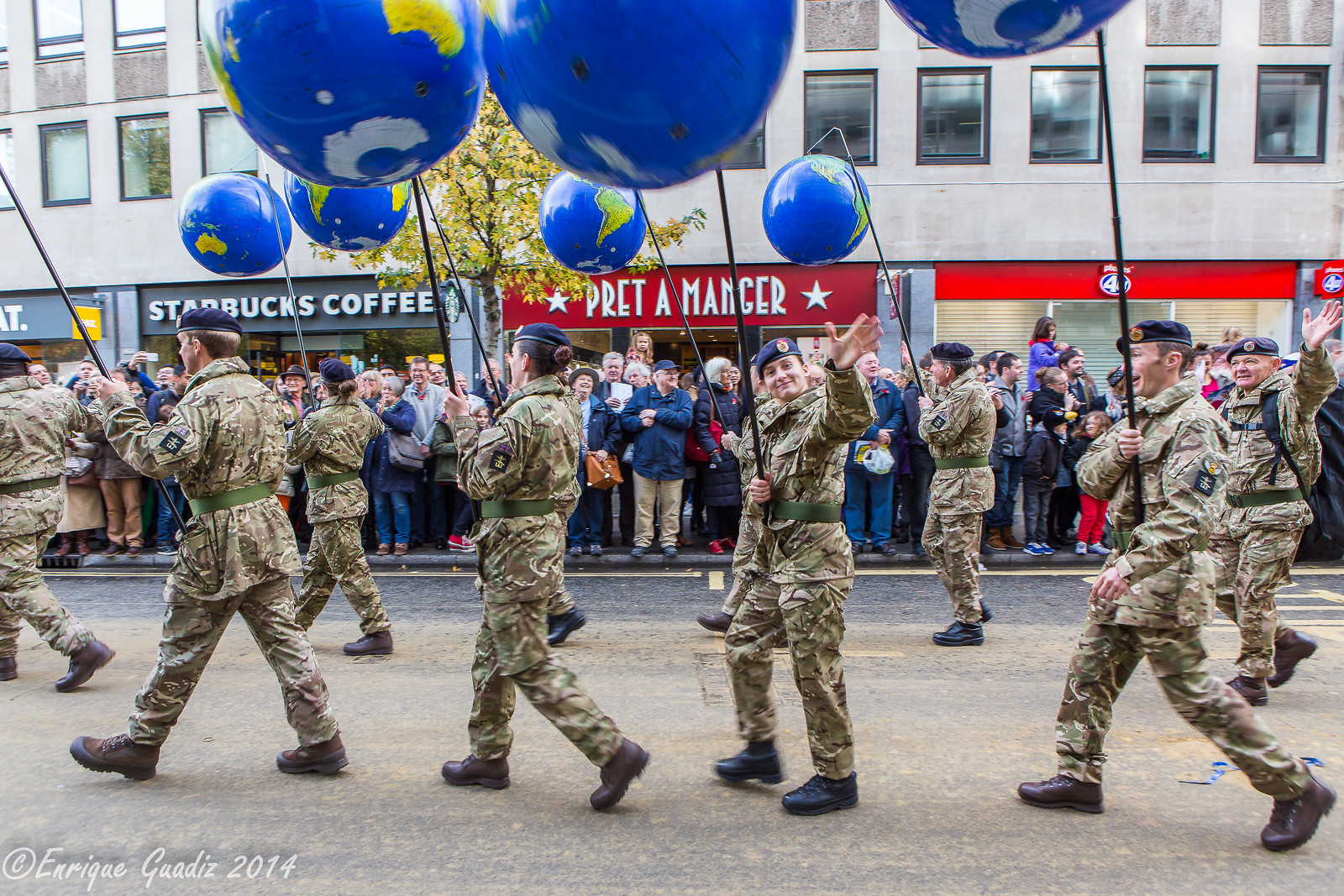The image captures a vibrant parade scene on a bustling street. The sidewalks are packed with a diverse crowd, standing shoulder to shoulder, some with children perched on their parents' shoulders, all observing the parade with a sense of excitement and wonder. In the middle of the street, uniformed men and women in military attire march in orderly lines. They wear camouflage-colored military pants and jackets paired with blue beret hats. Smiles light up their faces as they wave to the spectators. Each soldier carries a stick topped with a large blue globe, symbolizing the world. The atmosphere is bright and lively, amplified by the daylight and natural light flooding the scene. In the background, a large building with numerous windows stands tall, its ground level lined with storefronts, including recognizable names like Starbucks Coffee and Pret A Manger. The vibrant hues of the crowd and the orderly uniformity of the soldiers create a vivid contrast, making the scene both dynamic and captivating.